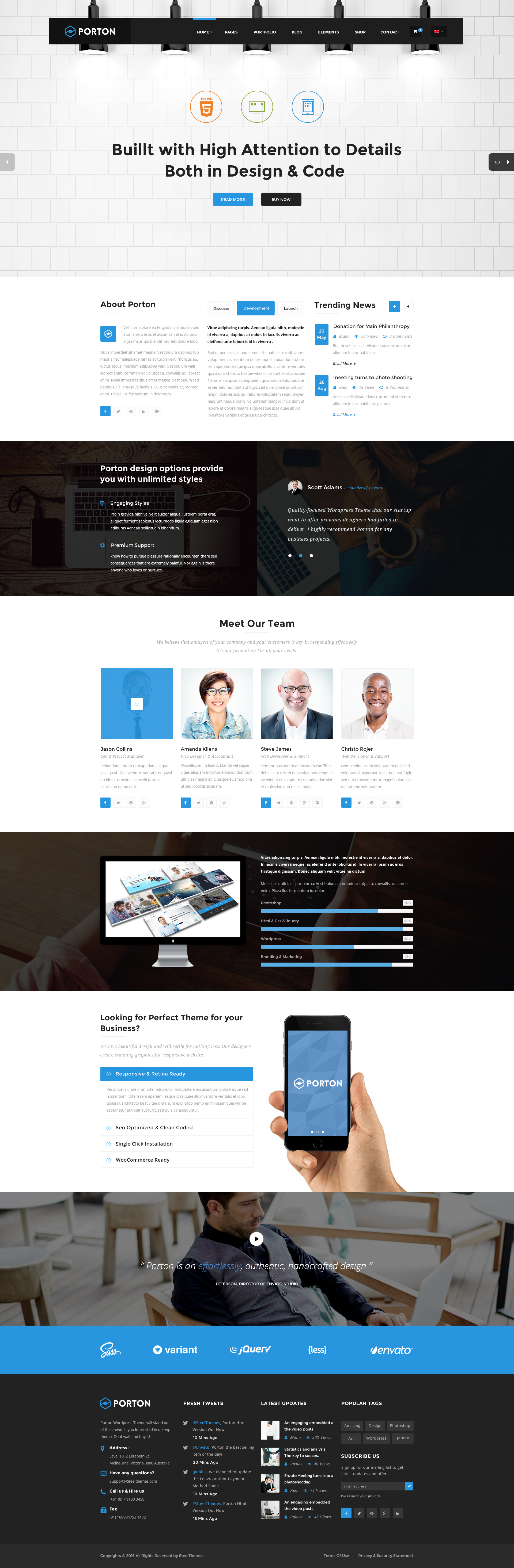**Website Overview**

The web page features a clean, white background with a gray header occupying the top one-fifth of the page. This header consists of a black menu adorned with white text, although the text is rendered too small to be read. The header also contains three icons, each with a distinctive color: orange, green, and blue. Below these icons, a bold statement in black reads, "Built with high attention to details both in design and code."

Below the header, the page includes two likely clickable areas, with one in blue and the other in black, each containing white text. Positioned on the far left of the gray header is a gray button, possibly a back navigation button. Conversely, a black button on the far right might function as a forward navigation button.

The main content area, which is white, immediately follows the gray header. This section displays some text, with specific portions emphasized within blue blocks, though the text is indistinct. Beneath this content lies a black block featuring white text, equally hard to decipher.

Further down, a white section labeled "Meet Our Team" displays profiles of four team members. Noteworthy is the absence of a picture for the first profile, typically the team's most crucial member, while the subsequent three profiles include images.

Continuing downward, there's another black block showcasing what seems to be web pages alongside a computer, accompanied by bar graphs positioned to the right. Beneath this block, a white section exhibits an image of a hand holding a phone, complemented by more text with certain parts highlighted by blue blocks.

The following segment features a picture of an individual working at a computer. Directly below this, a blue stripe displays several logos, which presumably belong to clients or partners. The page concludes with a probable contact information section, featuring typical details found on a website footer.